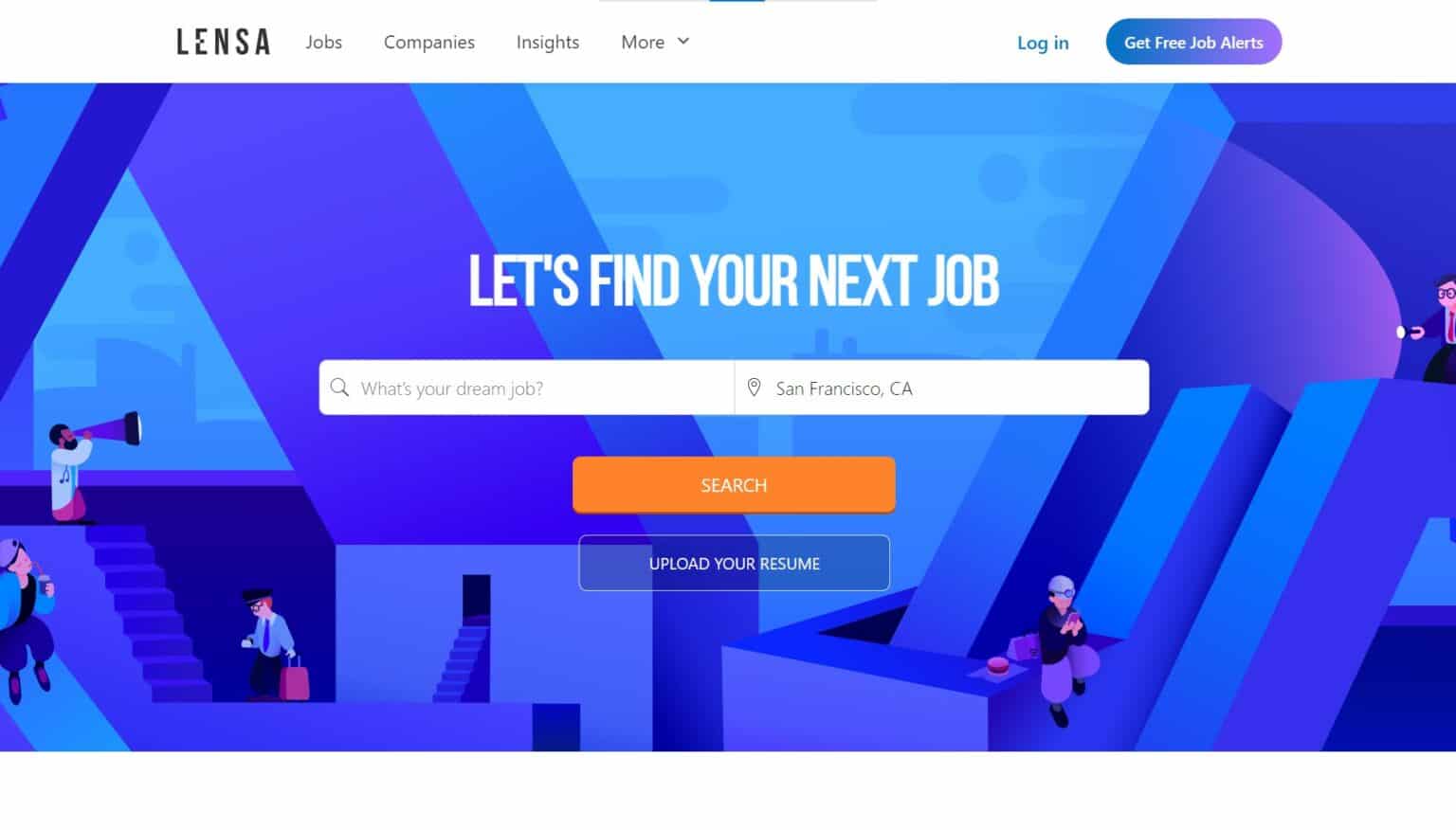The image is a rectangular graphic featuring a vibrant background composed of various geometric shapes in shades of bluish-purple. At the center of the image, a bold, white, all-caps text reads "LET'S FIND YOUR NEXT JOB." Directly below this text is a centered, thin white rectangular search bar. On the left side of this bar, there is a magnifying glass icon followed by the text "What's your dream job?" with a question mark. Adjacent to this, separated by a small line, is a location icon accompanied by "San Francisco, CA."

Beneath the search bar, there is a noticeable gap followed by an orange button with the white text "SEARCH." Directly below this button, another gap leads to a darker blue bar featuring the white text "UPLOAD YOUR RESUME."

The background further includes shaded areas depicting a cityscape. On the left side of the image, there are three figures: one is speaking into a megaphone, another is drinking a beverage, and the third is carrying a briefcase. On the right side, a person with round glasses peeks out from the edge, holding a flashlight. At the bottom right, a person is sitting on a ledge, eating lunch.